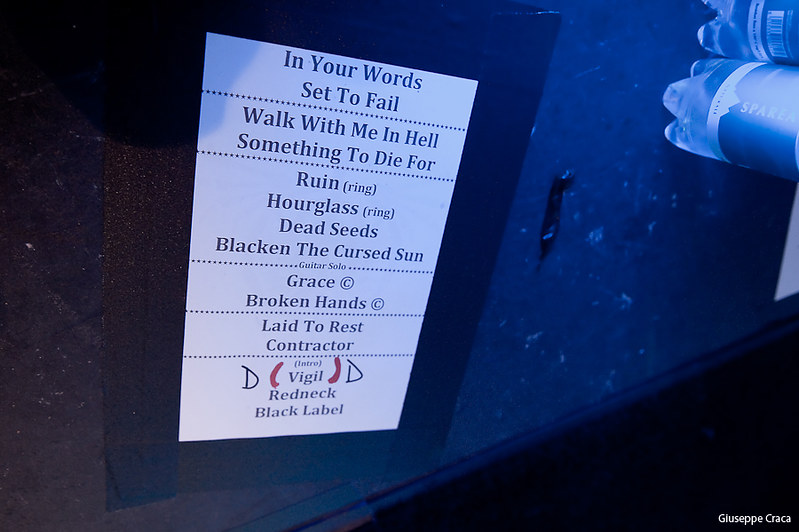The image features a dark background with a piece of paper attached to what appears to be a metal box, tilted sideways. The paper, which is white with black text, includes several song titles and annotations. The layout contains horizontal dotted lines separating the text segments. The text reads: "In your words, set to fail, Walk with me in hell, something to die for. Ruin (ring), Hourglass (ring), Dead seeds, Blacken the cursed sun." Below a dotted line labeled "guitar solo," the next section lists: "Grace ©, Broken hands ©, Laid to rest, Contractor." Further down, labeled as "intro," it states "Vigil" with red parentheses marked around it and flanked by a capital "D." The final lines read "Redneck" and "Black label." Surrounding the paper are a couple of soda bottles on the right side and a small black piece of something, possibly goo, on the metal surface.